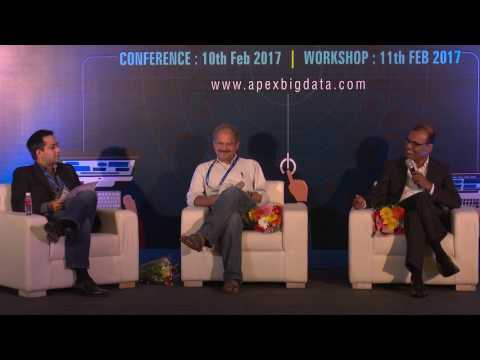In a spacious indoor conference setting, three men are seated in a row on plush, white easy chairs that are arranged across the center two-thirds of the stage. The backdrop features a navy blue panel with light blue text that reads "Conference: 10th February 2017" and "Workshop: 11th February 2017," as well as a website address "www.apexbigdata.com." Each participant is adorned with a lanyard, likely indicating their conference passes. The men on the left and right wear dark-colored suits, while the central figure dons a white long-sleeve shirt paired with green-blue pants and possibly sandals. Adjacent to each man is a colorful bouquet of flowers in yellow, red, white, and pink hues. The man on the right has his flowers on the chair to his right; the central man has his on the chair to his left; and the man on the left places his bouquet on the floor next to him, along with a bottle of water resting on the arm of his chair. The entire setup suggests a formal yet comfortable atmosphere, enriched by the vibrant colors of the flowers amidst the professional attire of the participants.